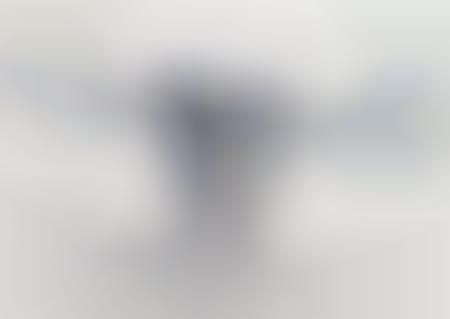The image is a small, rectangular, and blurry picture, predominantly featuring shades of gray and white. At the center of the image, there is a vague, dark, heart-shaped area, which is slightly darker than the surrounding palette and almost appears like a blackish blur. To the right center of this dark area, there is a subtle shape reminiscent of a fish fin. The bottom middle portion of the image is also noticeably darker than the rest. Overall, the image lacks distinct objects or text, making any specific setting or context indiscernible due to its low resolution and abstract quality.